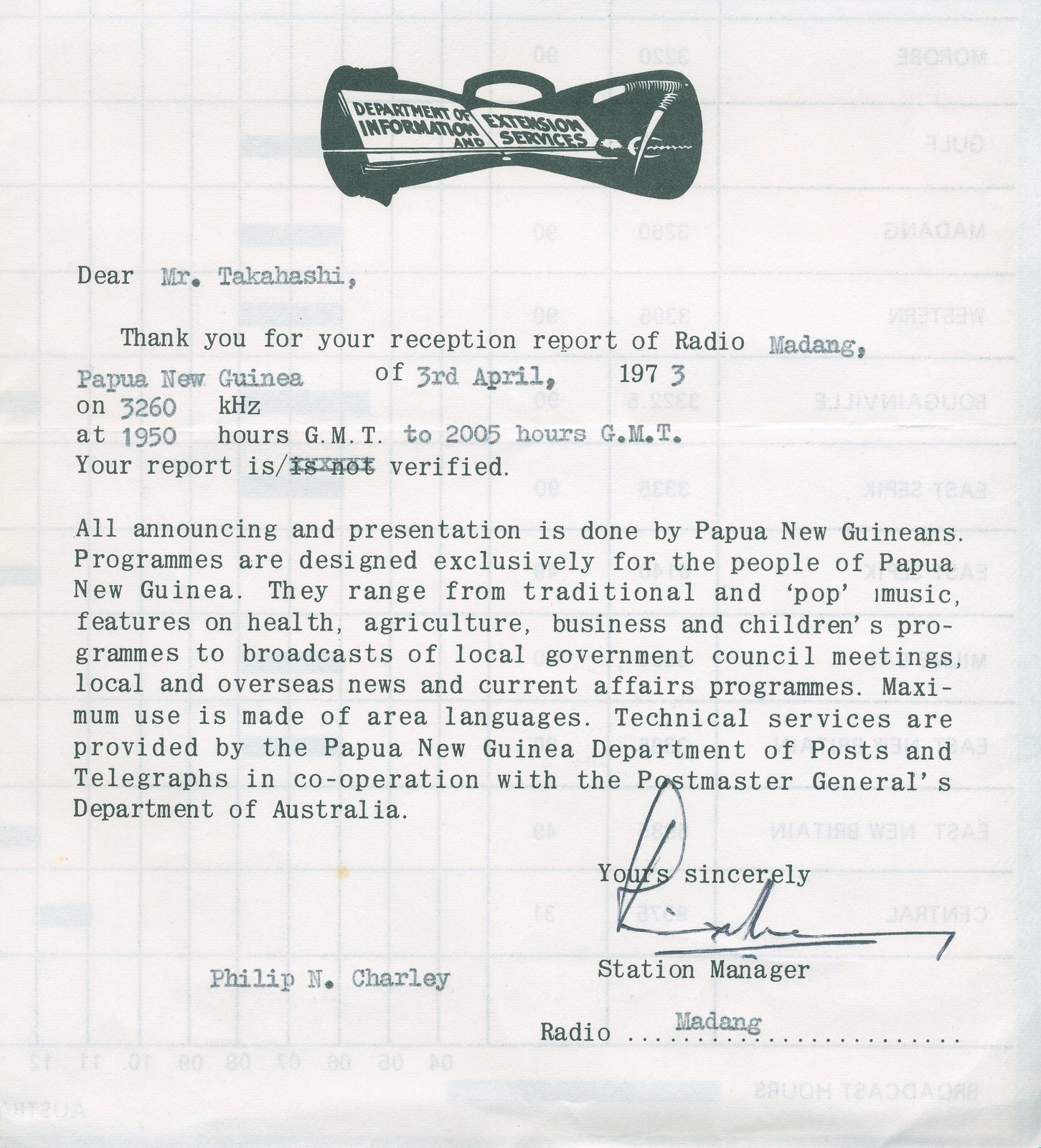This image displays a typewritten letter from the Department of Information and Extension Services, on a piece of white paper with faint blue graph lines in the background. At the top center of the letterhead, there is a black graphic resembling a suitcase or carry bag with a handle, which bears a white label that reads "Department of Information." Next to this label is another, smaller, unreadable white label. The letter reads in a black typewritten font:

"Dear Mr. Takahashi,

Thank you for your reception report of Radio Madang, Papua New Guinea of 3rd April, 1973 on 3260 KHz at 19.50 GMT to 20.05 GMT. Your report is [scratched out: is not] verified.

All announcing and presentation is done by Papua New Guineans. Programs are designed exclusively for the people of Papua New Guinea. They range from traditional and pop music, features on health, agriculture, business, and children's programs, to broadcasts of local government council meetings, local and overseas news, and current affairs programs. Maximum use is made of area languages. Technical services are provided by the Papua New Guinea Department of Posts and Telegraphs in cooperation with the Postmaster General's Department of Australia.

Yours Sincerely,"

The closing "Yours Sincerely" is centered over the lower right side of the report, followed by an unclear handwritten signature. Below the signature is the typed title "Station Manager," and further down on the lower left corner, the name "Philip N. Charley." In the lowest part of the right corner, the letter ends with the typed word "Radio," followed by a series of dots, and above these dots is the word "Madang."